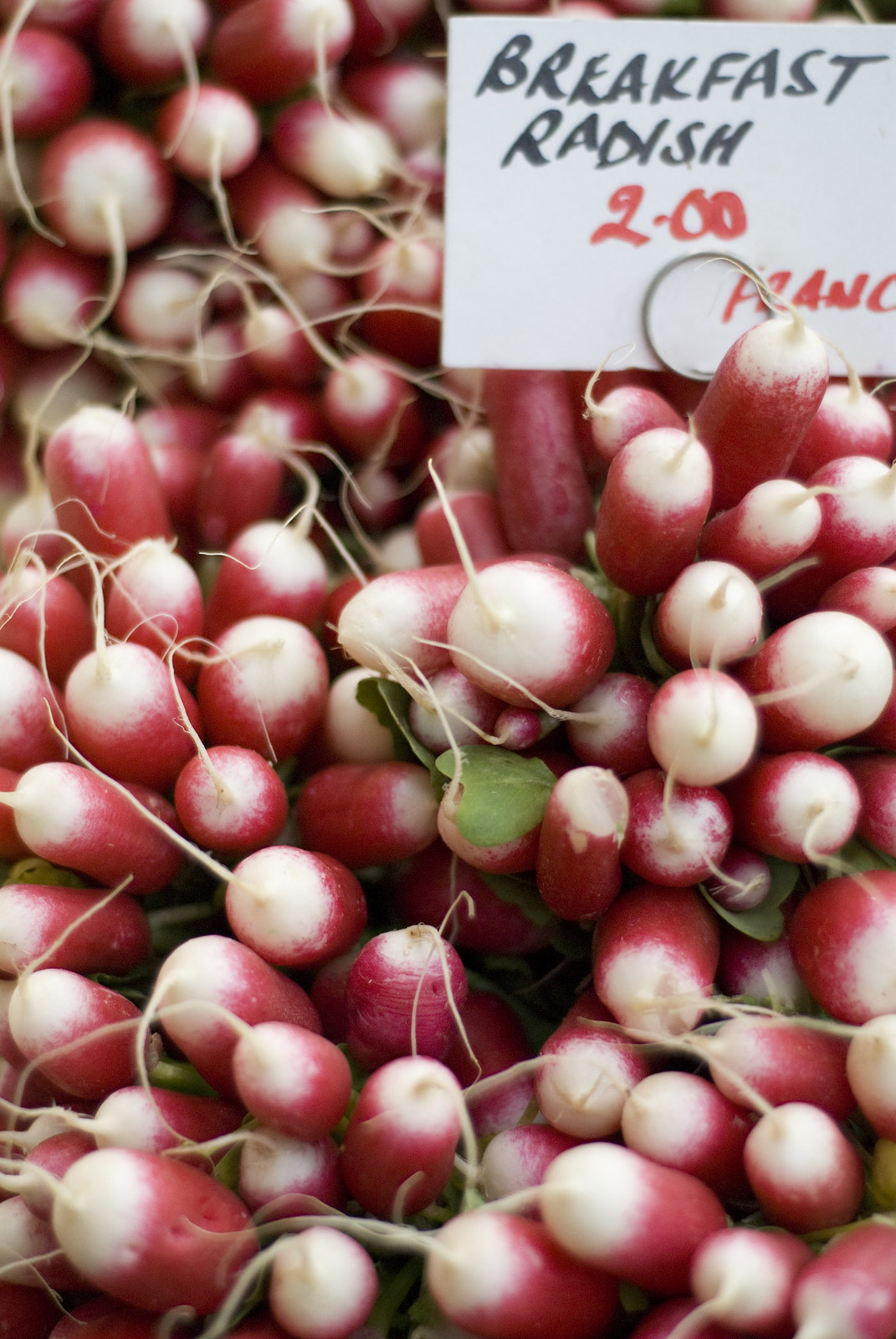The image is a rectangular composition filled with numerous radishes, primarily characterized by their white tops transitioning to pink bodies. Scattered throughout are some green leaves, adding a splash of color among the radishes. In the top right corner, there is a rectangular white label with text. The label reads "breakfast radish" in black letters and "2.00 franc" in red letters. The words "breakfast" and "radish" are centered on the sign, with "two dollars" below "radish" and "franc" starting just below the "0" in "2.00". The radishes appear to be freshly dug up, some with little thin strings still attached to them, giving a strong impression of freshness. The green leaves are more concentrated in the center and lower part of the image.